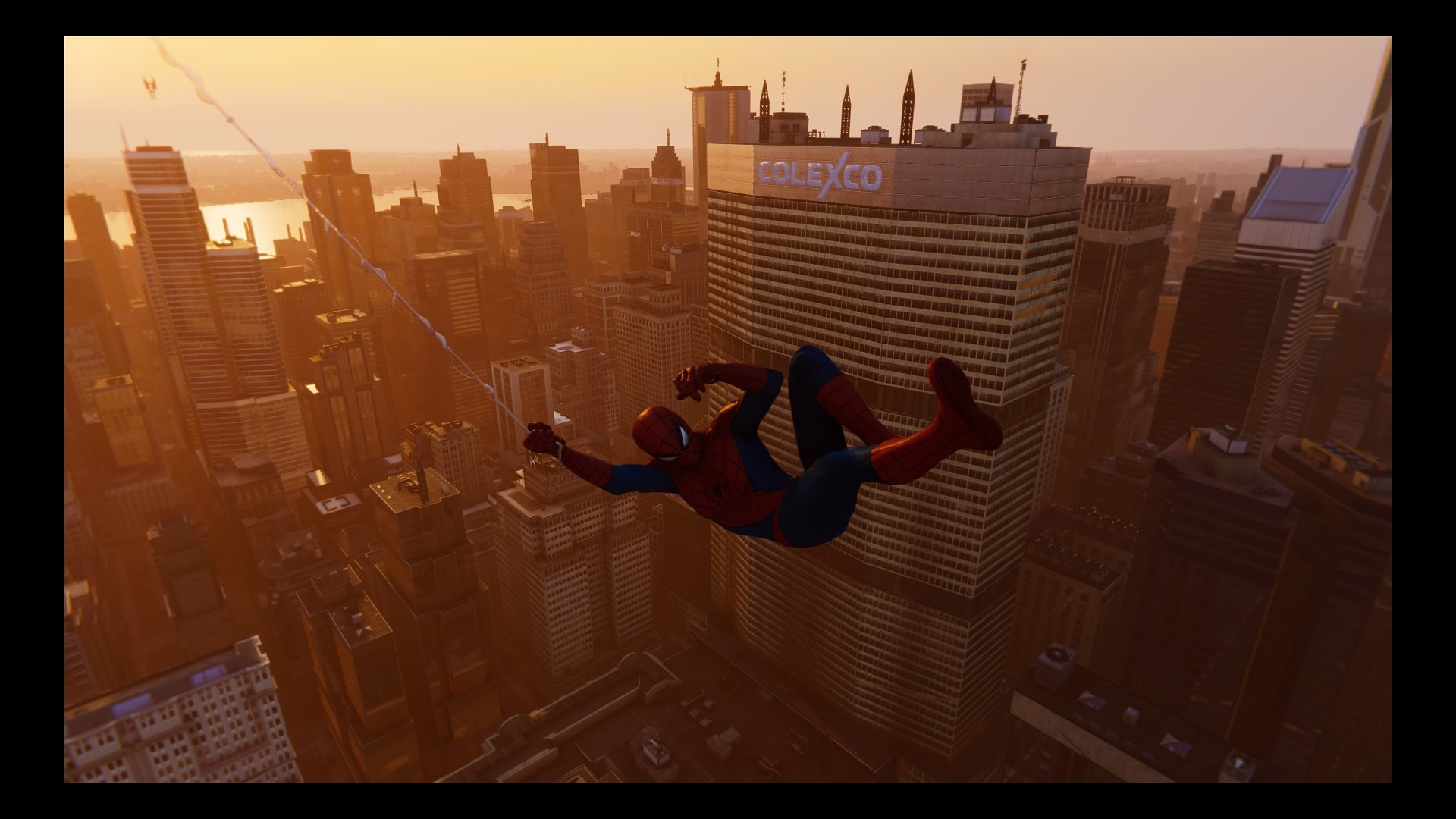In this vibrant image of Spider-Man, it appears to be a detailed scene likely taken from a movie. Spider-Man is positioned in the center of the frame, dynamically swinging through the air using a web that extends from his left hand towards the top-left corner of the image. His iconic suit is clearly visible, featuring red gloves, boots, and a mask with distinctive white eyes outlined in black. His chest, adorned with a spider emblem, along with his arms and legs, are clad in blue and red.

Spider-Man is captured mid-swing, with his legs projecting out in dynamic motion; one leg appears fully extended while the other is bent, suggesting he is in full swing to the right. The backdrop features a dense urban cityscape that strongly resembles New York City. Tall buildings and skyscrapers fill the scene, with a particularly prominent skyscraper at the center of the image, labeled with the name "COLEXCO" in uppercase letters at its top. There is a reflection of light glimmering on a body of water located in the upper left corner of the image, indicating a possible sunrise or sunset, adding a warm glow to this action-packed snapshot. This comprehensive scene beautifully encapsulates the essence of Spider-Man amidst the towering structures of the city he protects.